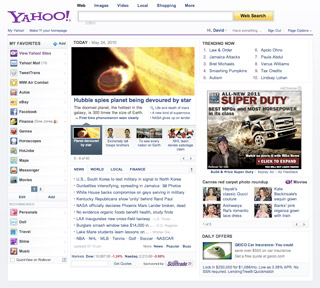This is a detailed descriptive caption for the provided image:

The screenshot is a small, zoomed-out capture of a Yahoo webpage. In the top left corner, the recognizable Yahoo logo is displayed in its signature purple color. Directly to the right of the logo, there's a horizontal navigation bar with various categories listed. Adjacent to these categories is a search bar accompanied by a button that could be green or yellow.

On the left side of the page, there is a column featuring icons paired with text labels, possibly representing different sections or services offered by Yahoo, with a total of around 15 items. Adjacent to this column, a real-time photo of outer space is prominently displayed alongside an article headline. Below this image, there are four smaller pictures, each with accompanying text, though the specifics are too small to discern.

Further down, additional text appears in blue, possibly hyperlinks or section titles. On the right-hand side of the page, another section provides a numbered list of items in blue text, though the details are too small to read clearly.

Beneath these sections, an advertisement for "Super Duty" is visible, featuring a man who resembles a personality known for doing "dirty jobs." The image includes a truck, seemingly attempting to navigate through dirt or mud.

Lower still, there are photos of four women, each neatly aligned in a single section, accompanied by blue titles next to each image. At the bottom of the screenshot, there is likely another advertisement, possibly for a tech product, with text both beside and beneath the image.